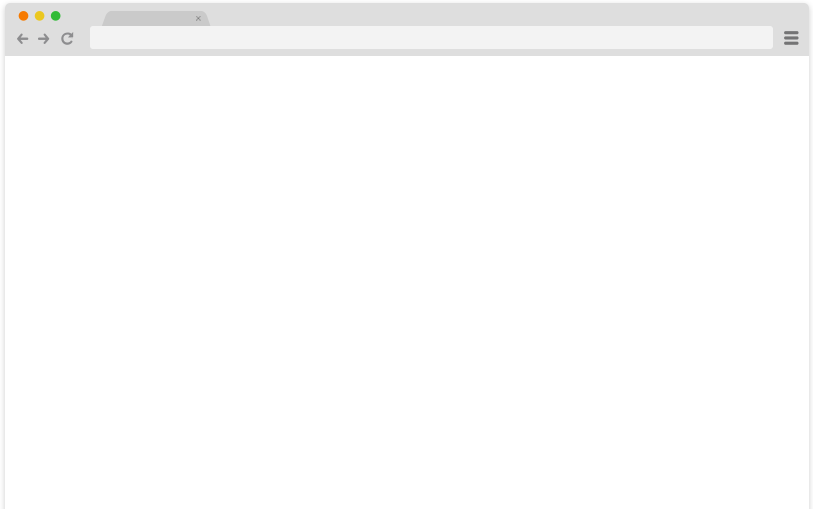The image depicts a minimalistic webpage displayed within a web browser interface against a white background. The browser window showcases no content or text. The frame of the browser has a light gray perimeter, with the bottom edge seamlessly blending into the white background of the webpage. 

On the left and right sides of the browser frame are two thin vertical gray lines, and at the top is a slightly thicker gray border. In the upper left-hand corner of this border are three sequential dots in red, yellow, and green, commonly associated with window control buttons, possibly indicating the Opera browser interface, though this is not definitively confirmed.

Next to these dots is a darker gray tab featuring a small 'X' for closing the tab. Below the tab area, navigation icons are displayed: a back arrow, a forward arrow, and a refresh icon, all in a darker shade of gray. Adjacent to these icons lies a light gray search bar. Finally, at the top right corner of the browser frame, there are three horizontal lines in gray, typically representing a menu or settings option.